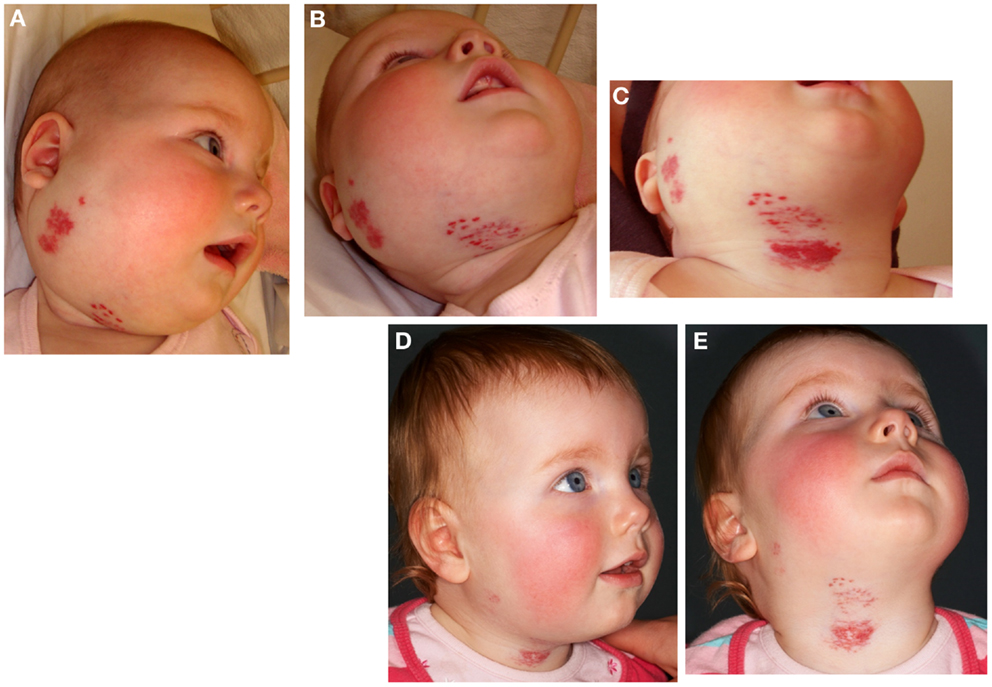The series of five photographs depicts the progression of healing in a baby with noticeable facial and neck rashes. Labeled A through E, the images transition from left to right on the top row and from left to right on the bottom row. 

In Photo A, positioned at the top left, we see the right side of a young child's face with a severe bright red rash and swelling extending from the right cheek to the ear and neck. The background is mostly white, probably due to pillows. The baby has a pale complexion and minimal hair.

Photo B, the middle image on the top row, offers a lower angle view under the baby's chin, highlighting the extensive rash below the right ear and towards the neck.

Photo C, at the top right, provides an even lower perspective further under the chin, focusing on the bright red splotches beneath the baby's neck.

Moving to the bottom row, Photo D, to the left, captures the same child at a later stage. The baby appears older with more hair and a noticeable reduction in the rash and swelling. The background is now dark gray. The rash is still present but substantially healed.

Finally, Photo E, to the right of D, shows a similar timeline where the baby’s head is tilted upwards, revealing the residual splotches on the neck. The child, now older, has more hair and the rash is significantly diminished.

Together, these images document the initial severity and subsequent healing of the baby’s rash over time, highlighting the changes in appearance and background between the earlier and later stages.